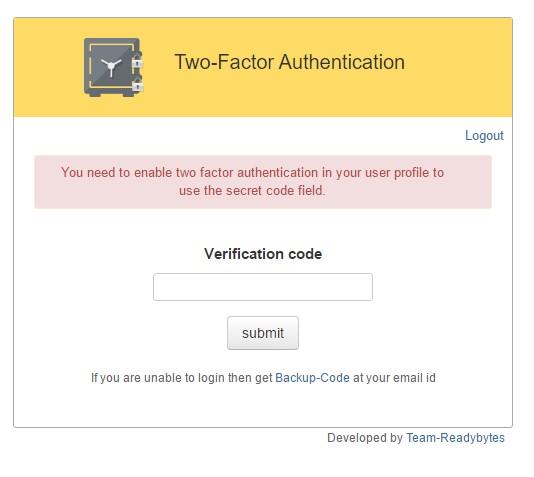This image is a screenshot of an interface for enabling two-factor authentication. It features a square design bordered by a light gray edge. At the top, there's a yellow bar with an icon on the left depicting a safe, complete with a circular dial and two locks. This icon symbolizes the security feature being described. 

To the right of the yellow bar, black text reads "Two-Factor Authentication."

Below this section is a larger box with a white background. Toward the top right of this box, there is a blue "Log Out" link. Beneath the "Log Out" link is a light pink box with red text stating, "You need to enable two-factor authentication in your user profile to use the secret code field."

Further down, bold black text reads "Verification Code," followed by an input field for the user to type their code. Below this input field, there is a "Submit" button.

At the very bottom of this main box, there is a line of text in black that advises users who are unable to log in to obtain a backup code via email. The phrase "backup code" is clickable and appears in blue.

At the very bottom of the interface, outside the main box, there's a small note in black text reading "Developed by," followed by "Team ReadyBytes" in blue ink. The word "ReadyBytes" is spelled as R-E-A-D-Y-B-Y-T-E-S.